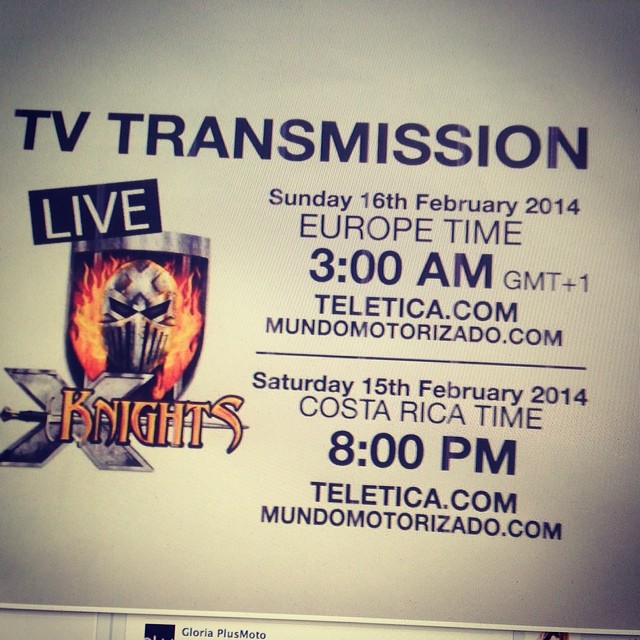This image displays a digital advertisement for a TV transmission of a show titled "LIVE KNIGHTS." The advertisement, captured from a computer screen, features a knight's helmet emblem with flames around it, above a giant "X" and a sword that intersects with the "X". The word "KNIGHTS" is inscribed along the blade of the sword. The ad announces live broadcast times as follows: Sunday, 16th February 2014 at 3:00 AM European time (GMT+1) and Saturday, 15th February 2014 at 8:00 PM Costa Rica time. Accompanying these details are two website addresses: teletica.com and mundomortizarazo.com. The image quality is not optimal, suggesting it was taken with a camera aimed at a computer screen.